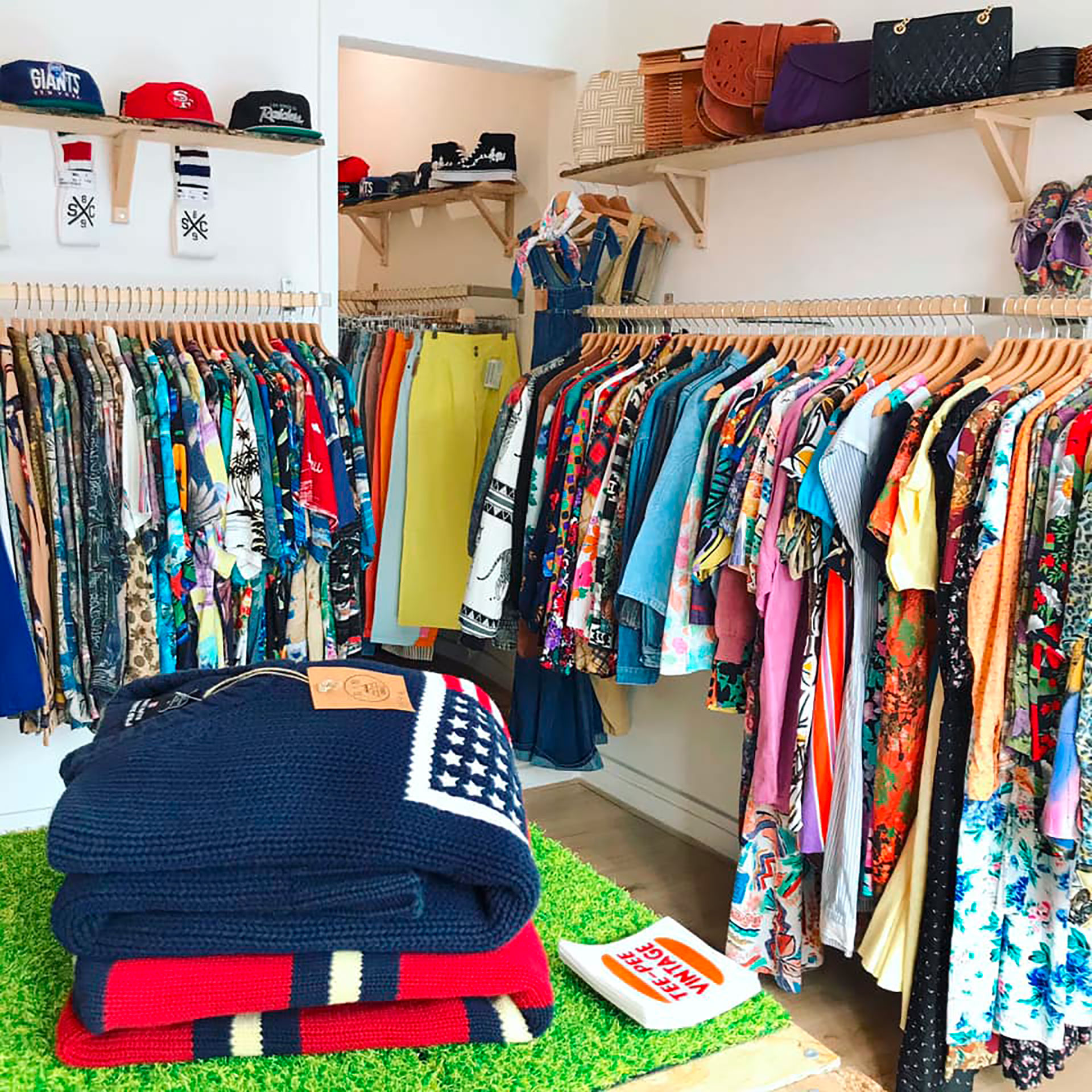This image captures a well-organized display inside what appears to be a clean and inviting thrift store. Brightly colored shirts and dresses with tropical designs, featuring palm trees and flowers, dominate the scene. These garments hang neatly on wooden racks along both white walls, and some denim clothing and overalls are also visible. In the foreground, there are two folded sweaters on a table with a green AstroTurf covering. One sweater is blue with part of an American flag visible, while the other is red with blue and white stripes. Above the racks, shelves contain various accessories, including several hats representing different sports teams like Giants, SF for San Francisco 49ers, and Redskins. Additional shelves display purses and shoes. A doorway leads to a secondary room where more skirts or pants hang. The attention to detail and variety in this thrift store make it a visually appealing space.